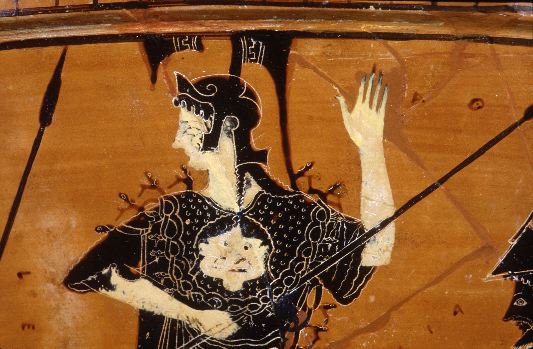This close-up photograph captures a section of ancient, weathered Greek black-figure pottery, likely made of wood, but traditionally possibly ceramic. The piece features a detailed, albeit somewhat distorted, drawing of a military figure, possibly a soldier or a deity such as Athena. The figure is depicted in a traditional black-figure style against a red background, dressed in black armor including a helmet and a tunic. The individual holds a spear with one arm raised, and the other arm bent towards their stomach. An emblem resembling a mashed or face is present on their chest. Intriguingly, parts of another figure are visible, including a spear tip and a face wearing a Spartan helmet, hinting at a larger, more complex scene.